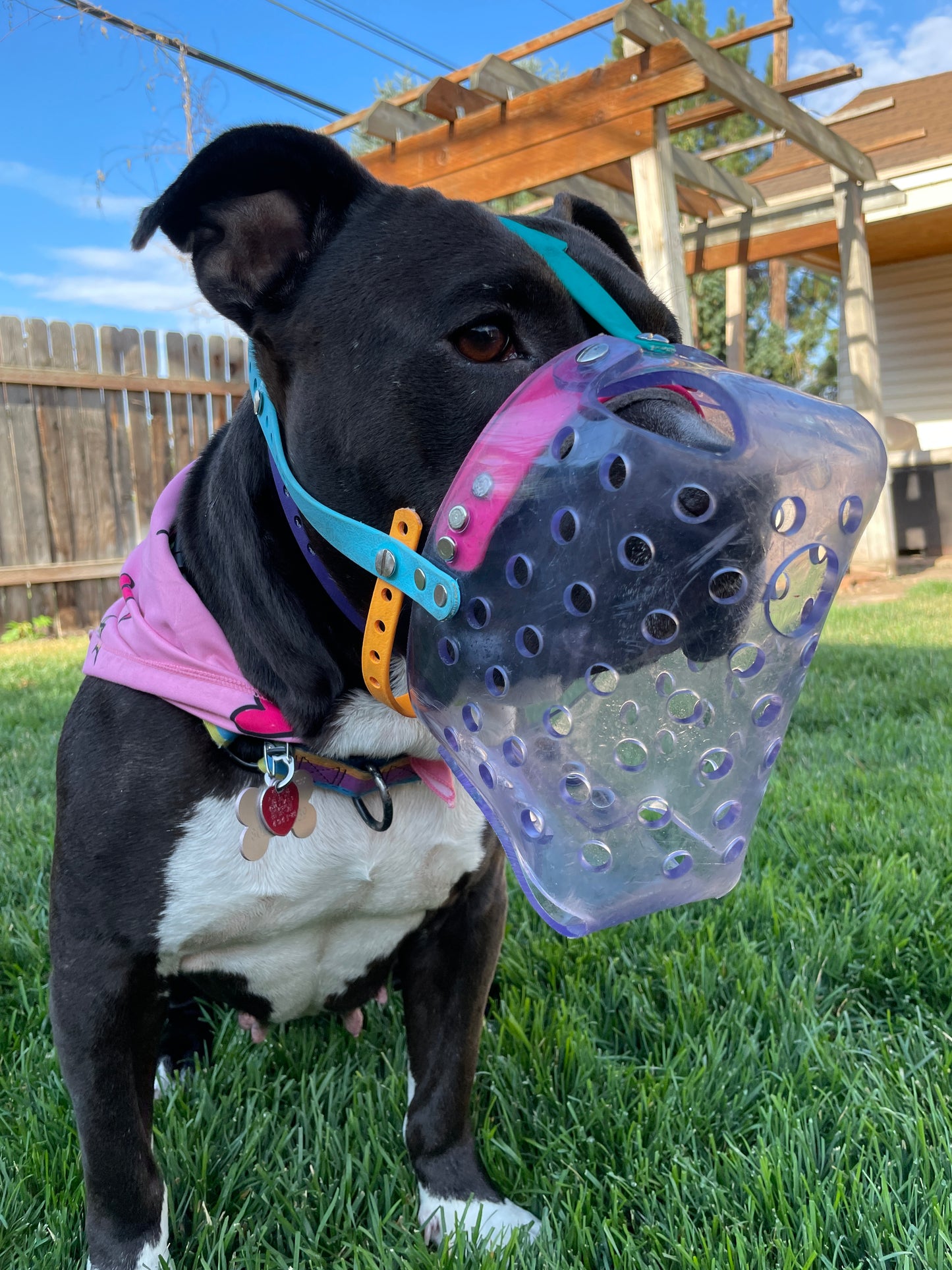In this detailed daytime photo set in a backyard, a black pit bull with a distinct white chest and white markings on the bottom of its two front legs is the focal point. The dog is adorned with a pink bandana around its collar and a clear, box-shaped plastic mouth guard, secured by colorful straps in light blue, bright orange, and hot pink. The dog's head is also topped with a small pink cap. Surrounding the dog, the backyard features a lush grassy area with a wooden fence to the left and a house with white siding and a brown roof to the right. In front of the house, there is a booth with a brown top. The photo is taken under a blue sky scattered with white clouds, enhancing the tranquil outdoor setting.